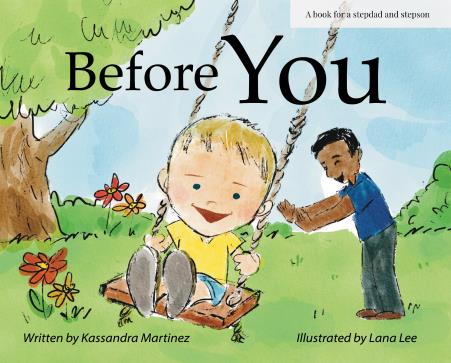The illustrated front cover of the book, written by Cassandra Martinez and illustrated by Lena Lee, portrays an engaging scene designed for a story about the relationship between a stepdad and his stepson. The central text "Before You" is prominently displayed in a large serif font, capturing immediate attention. A white rectangular banner in the top right corner indicates the book's theme, "A book for a stepdad and stepson."

In the image, set against a bright blue sky backdrop, a father figure with brown skin, wearing a blue shirt, dark teal/black pants, and brown shoes, pushes a young boy on a wooden swing suspended by thick ropes. The man has short black hair and a big smile, joyously extending his arms to push the swing. The boy, featuring lighter, tan/peachy skin, blonde hair, and a yellow shirt with blue shorts, is equally delighted, holding tightly to the swing's ropes and smiling broadly.

The scene is set in a lush yard with a large tree, possibly a maple, on the left side. Brown trunk and green leaves adorn the tree, while the ground is covered in green grass peppered with red and orange flowers, adding vibrant colors to this lively and heartwarming illustration.